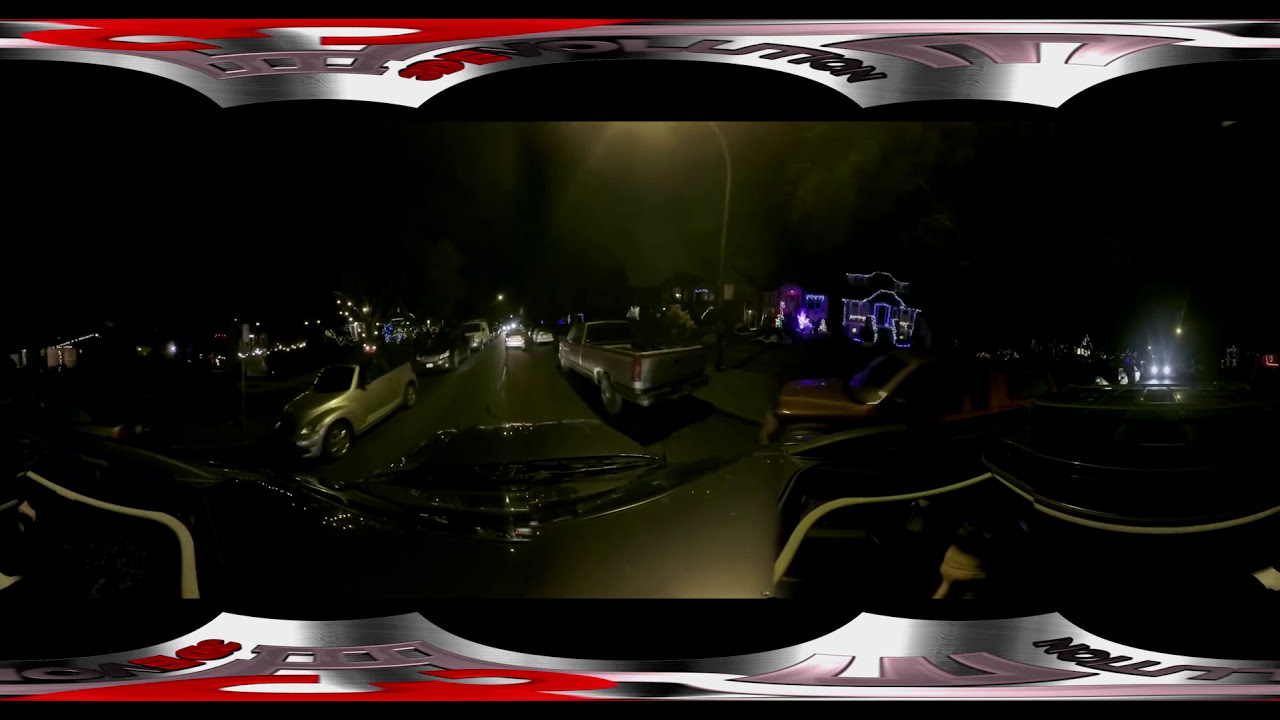The image depicts a nighttime suburban scene, as viewed through a car window. The image has a warped and curvy appearance, suggesting it might have been taken with a 360 camera, which distorts the scene into a flattened, panoramic view. The top and bottom sections are framed by a decorative gray and red design, partially overlaying text that seems to spell out "O-L-U-T-I-O-N." This provides the impression that the photograph was taken from inside a vehicle, possibly a silver car that is driving down the road.

The scene outside includes a blacktop road bordered by parked vehicles on both sides. Some cars have their headlights on, hinting at activity despite the late hour. A pole, with light radiating from an unseen streetlight, adds a soft amber glow to the surroundings. Houses line both sides of the road, one of which stands out for its festive decorations, adorned with white Christmas lights around its structure and blue glowing lights in the yard. This house, positioned to the right within the frame, suggests a holiday season atmosphere. The predominant colors in the image are black, off-olive green, red, gray, and silver, with illuminated areas cutting through the otherwise dark scene. No people or animals are visible, but the presence of lit houses and moving cars indicates an inhabited, lively neighborhood.